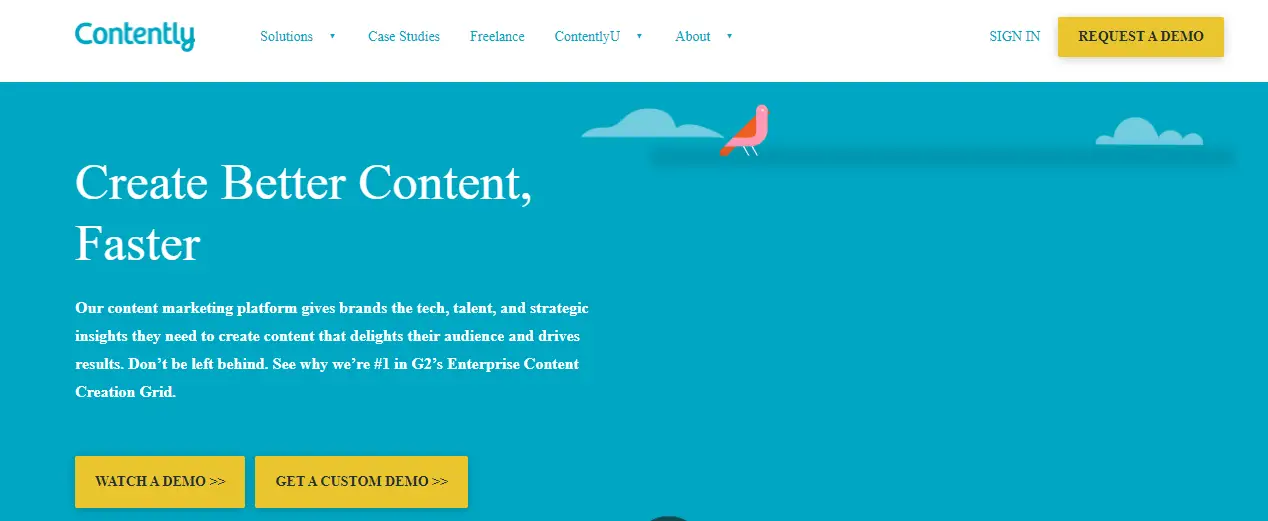The image features a rectangular layout approximately 2.5 to 3 times wider than it is tall. 

At the very top, occupying about 20% of the height, is a horizontal white background displaying the company’s branding elements. On the left, there’s a light blue company logo featuring the word "Contently," with a distinctive cursive "Y." To the right of the logo, an aligned menu displays navigation options in light blue text: Solutions, Case Studies, Freelance, Contently You, and About. On the far right, there is a "Sign In" option, followed by a bright yellow button labeled "Request Demo" in black text.

Below this header, the main banner spans the rest of the image. The background is predominantly a matching light blue, depicting a blue sky with a few slightly lighter blue clouds. Toward the upper right, a stylized bird with pink and red wings adds a touch of visual interest. 

On the left side of the banner, white text stands out prominently. In very large font, it reads "Create Better Content," with each word's first letter capitalized. Directly below, the word "Faster" is also capitalized and in large white text. Underneath these headlines, a smaller paragraph provides a brief description of the site’s offerings. The section concludes with two call-to-action buttons: one to "Watch a Demo" and another for "Get a Custom Demo."